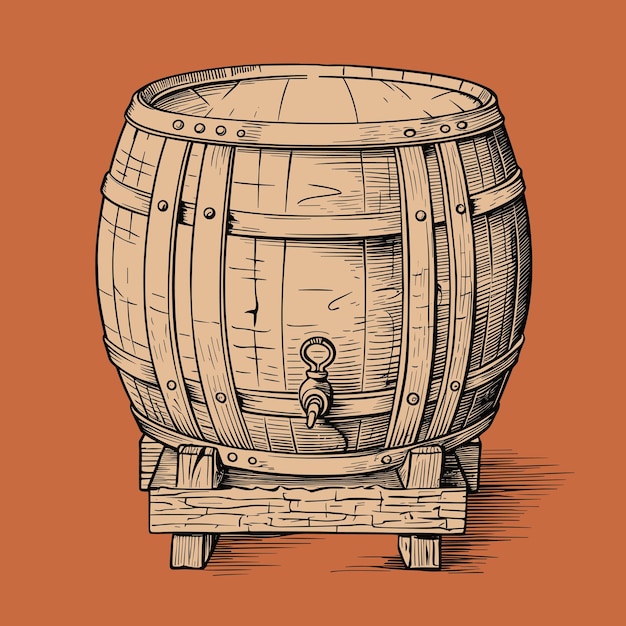The image portrays a cartoonish drawing of a short and wide wooden barrel, resembling those used for whiskey or wine. The barrel is made of tan-colored wood planks and features a closed top. It is secured with two horizontal bands around the midsection and two vertical bands on the sides. A spigot with a pole lever, encased in a circular ring, protrudes from the front, indicating that it can be used to dispense liquid into a glass or cup. The barrel is propped up on a light-colored wooden stand, possibly made from two-by-fours, which adds elevation. The entire setup is set against a solid burnt orange background with black line work indicating the ground beneath the stand, adding to the overall rustic charm.